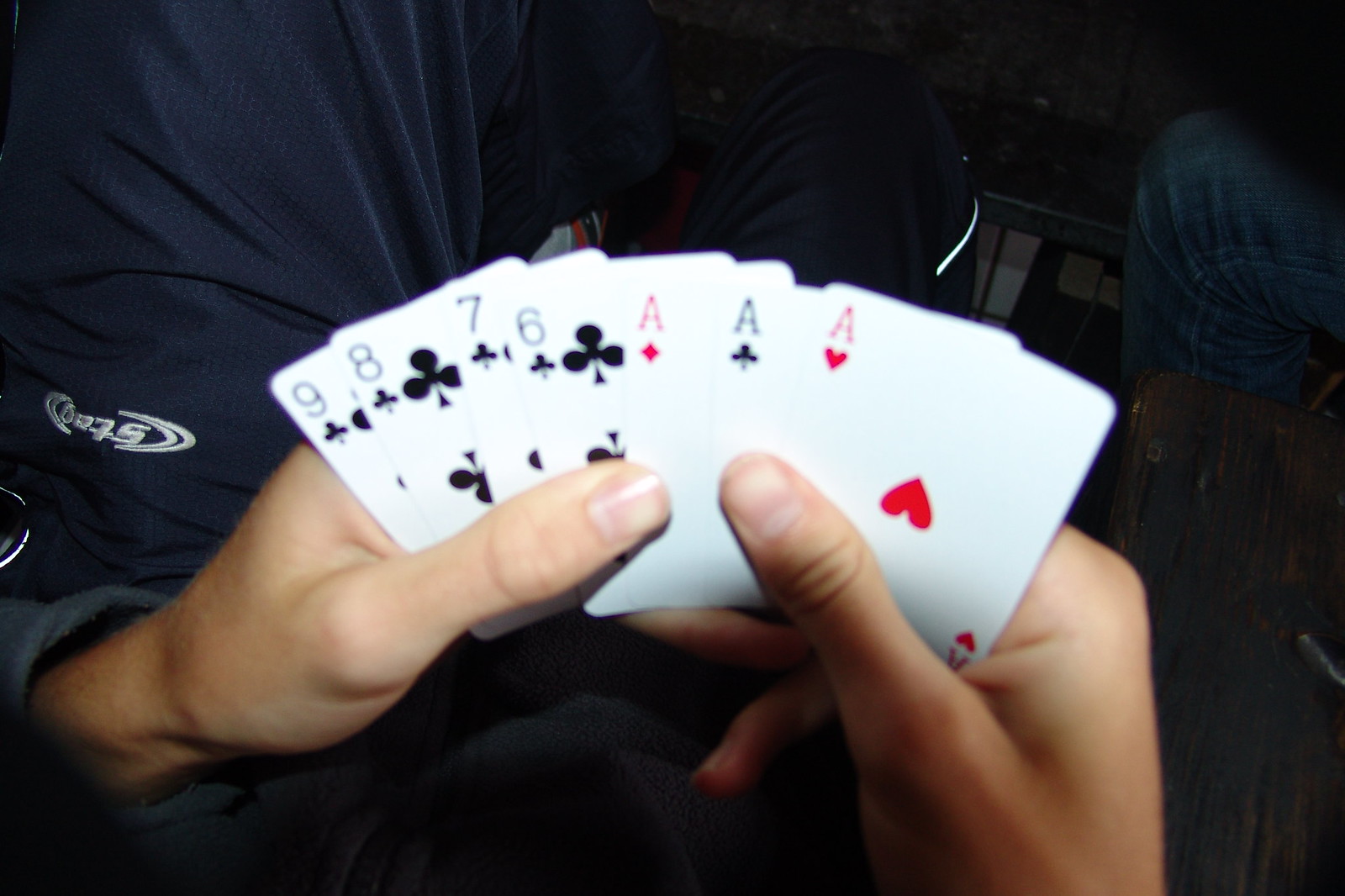A person is shown holding a hand of seven playing cards, arranged fan-like, with their hands positioned near their chest. The visible cards include a sequence of four clubs: nine, eight, seven, and six, along with three aces: ace of diamonds, ace of clubs, and ace of hearts. The individual appears to be seated, wearing a gray sweater, and perhaps blue sweatpants or joggers, indicated by the visible sleeve and clothing. To the right, another person, clad in jeans, is partially visible, hinting that he might be participating in the same card game. This compelling spread of cards suggests the game could be poker, albeit with an unconventional number of cards, or possibly another card game such as Go Fish.